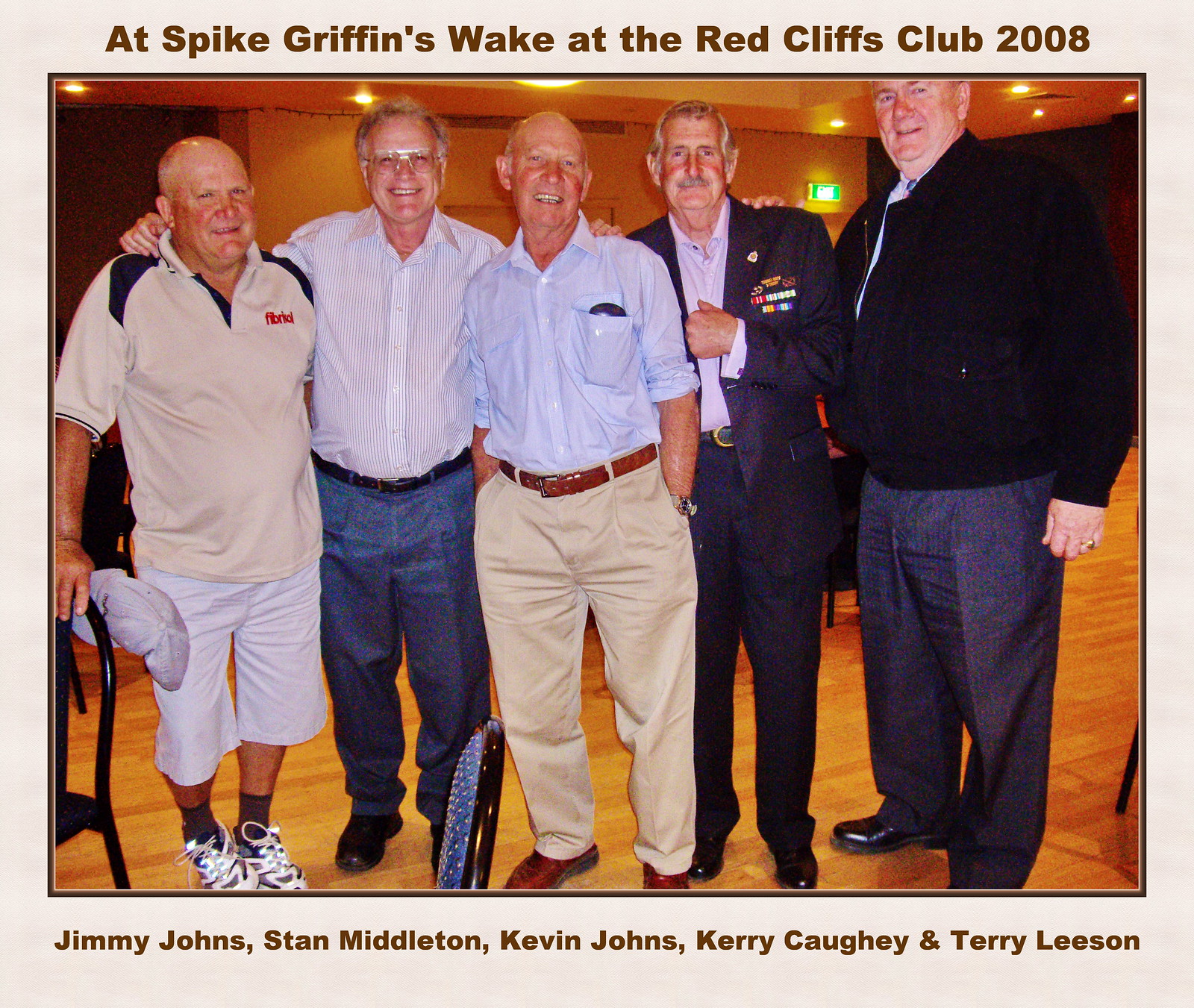The photograph is set against a light beige background and framed by a thin brown border. At the top, in brown letters, it reads "At Spike Griffin's Wake at the Red Cliffs Club 2008." The picture features five older men standing, smiling, and posing for the camera, with some of them having their arms around each other. They are arranged against what appears to be the interior of a banquet hall or restaurant, with visible tables, chairs, recessed lighting, and a green exit sign over their shoulders. 

From left to right, the first man is bald, wearing a beige polo shirt with black shoulder accents, khaki shorts, brown socks, and tennis shoes. The second man, with gray hair and glasses, sports a blue and white striped shirt, jeans, a belt, and dark shoes. The bald third man is dressed in a light blue button-down shirt, a brown belt, khaki pants, and brown shoes, with his hands in his pockets. The fourth man, who has gray hair and a gray mustache, wears a blue shirt with a blue suit adorned with medals. The fifth man dons dark slacks, a black jacket, and a button-down shirt. 

Beneath the photograph, in smaller brown letters, the caption names these men as Jimmy Johns, Stan Middleton, Kevin Johns, Kerry Caughey, and Terry Leeson.